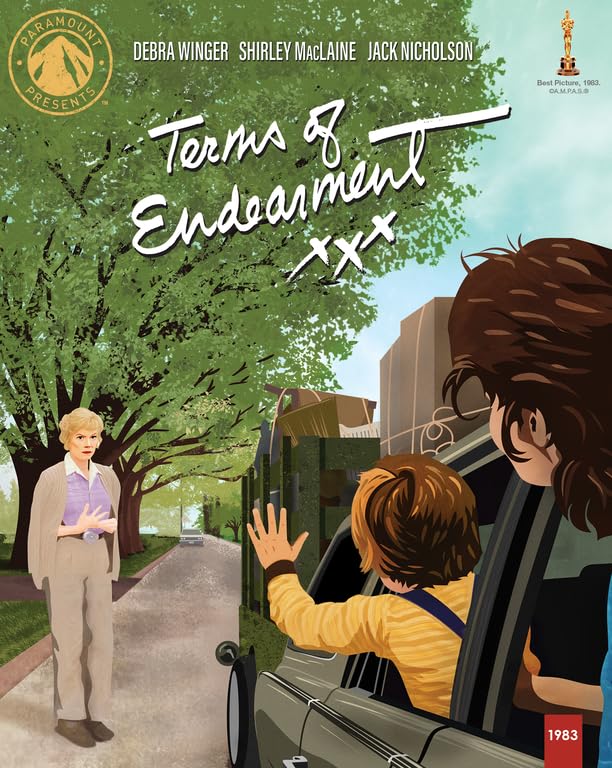The illustrated movie poster for "Terms of Endearment" features the title prominently in white text near the top, just below the names of the starring actors: Debra Winger, Shirley MacLaine, and Jack Nicholson. Above these names, a gold "Paramount Presents" logo is displayed. An Oscar statuette in the top-right corner signifies the film's Academy Award win. The main illustration depicts a scene with a car driving away on a road lined with trees. The car, seen partially from the side, is packed with luggage and possibly towing a trailer. Inside, a child is waving from the backseat, while another person's head, presumably Shirley MacLaine's character in khaki pants, a khaki cardigan, a blue shirt with a white collar, and blonde hair, is seen peeking out of the passenger window, though not waving. Standing on the roadside, also dressed in khaki pants, a khaki cardigan, a blue shirt with a white collar, and with blonde hair, is a woman who looks like Shirley MacLaine. At the bottom of the poster, within a red square, the year "1983" is marked in white.